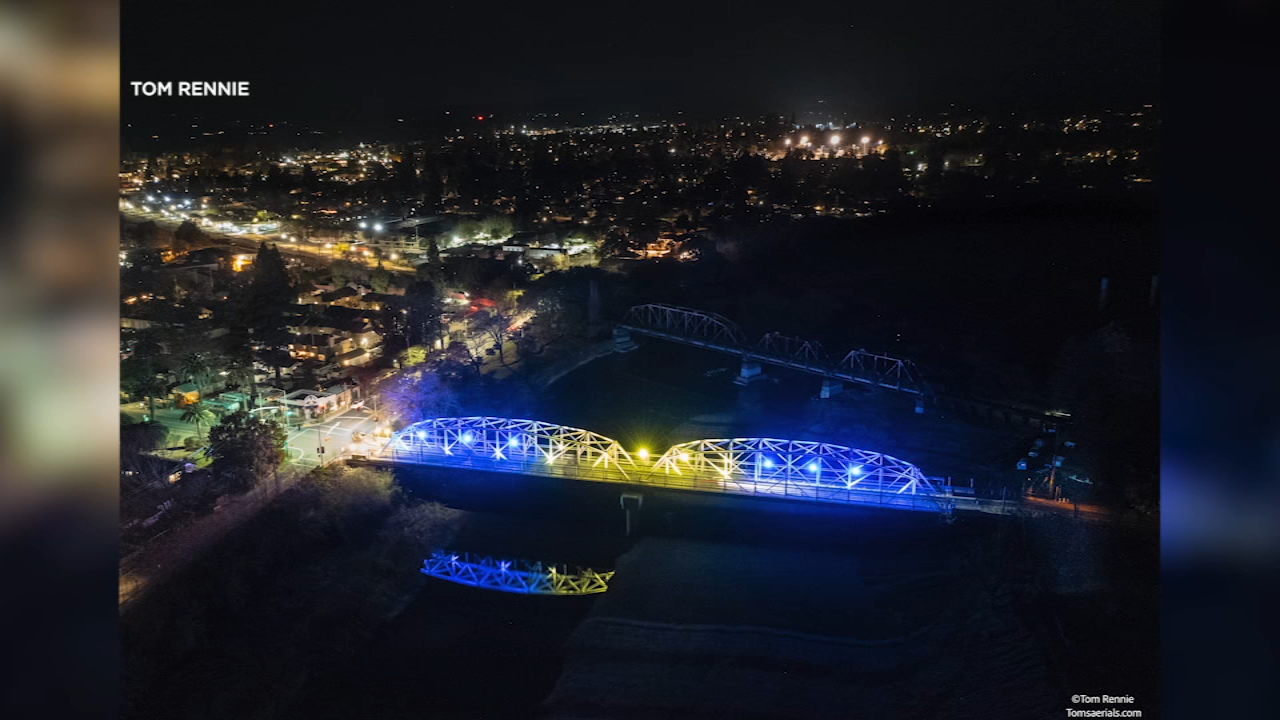This is an aerial view photograph of a city at night, prominently featuring a waterway and two bridges. The most striking of the bridges is illuminated with vibrant blue and yellow lights, creating a dome-like pattern across its expanse. The bright lights extend from the left, where a roadway exits the bridge with an especially bright light, across the center with yellow illumination, and to the right side with more blue lights. The reflections of these lights glisten on the black surface of the water below. To the left and right in the distance, city lights are visible, suggesting a sprawling urban expanse. The cityscape is characterized by numerous buildings and structures, none of which are particularly tall, their lights dotting the landscape. Streets crisscross through the city, with the headlights of cars adding to the glittering scene. In the background, another bridge can be seen, but it is not illuminated, offering a stark contrast to the brightly lit main bridge in the foreground.